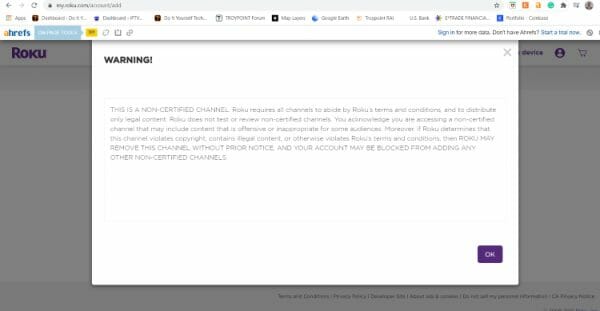The image depicts a web browser interface that is notably blurry, making it difficult to discern specific details. At the top, the address bar contains a typed URL, accompanied by navigation icons, including a back button, a refresh button, and approximately seven additional icons to the right. Below the address bar is a bookmark bar featuring around a dozen bookmarks, although their identities remain indistinct. Beneath the bookmark bar is a tab labeled "HREFS." The main content area displays a mix of elements, including a blue box and a yellow box, as well as some icons, one resembling an attachment icon. A prominent white pop-up window with a warning sign in bold black capital letters is also visible, featuring an 'X' symbol for closing the window. The pop-up contains a paragraph that begins with "NON-CERTIFIED CHANNEL" in capital letters, though the remainder of the text is too small to read. At the bottom of the pop-up window is a purple box with the word "OK" centered within it.